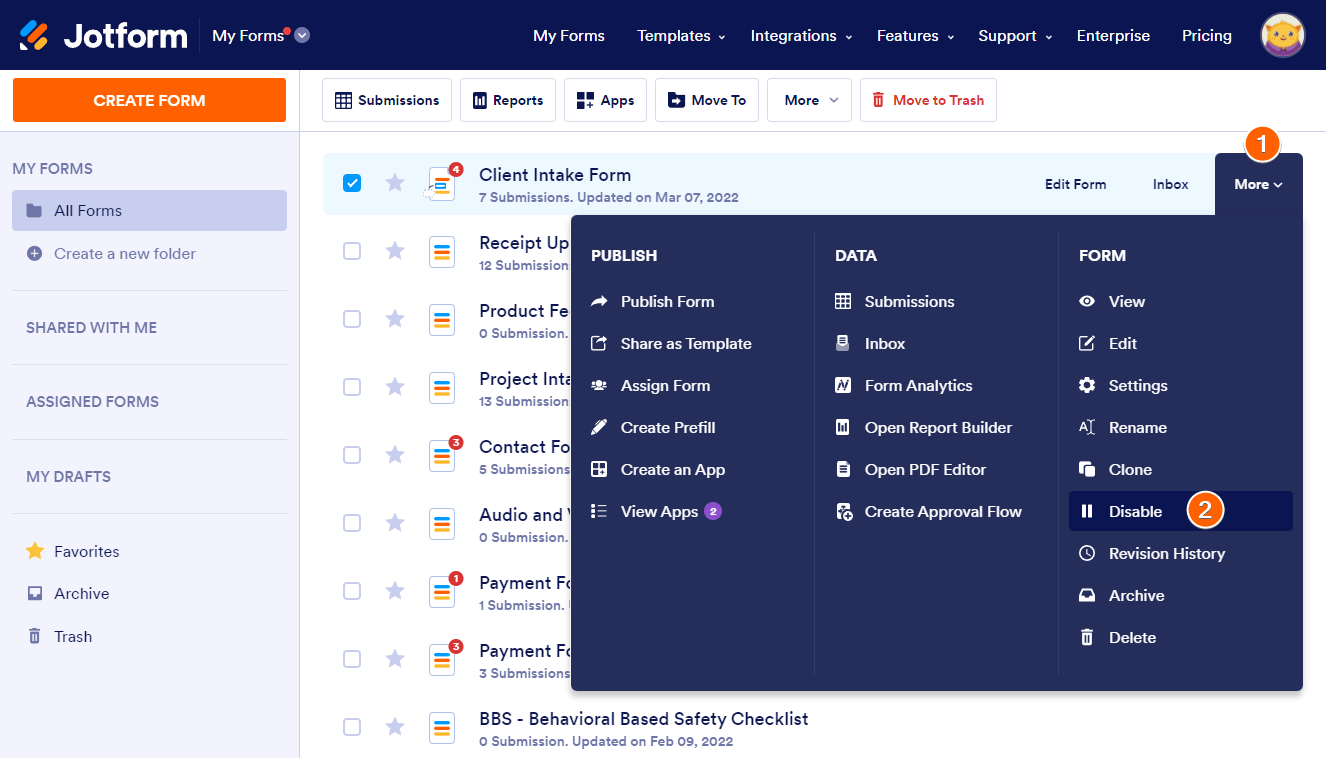The image depicts the JotForm website interface, prominently featuring several navigation tabs at the top: "My Forms," "Templates," "Integrations," "Features," "Support," "Enterprise," and "Pricing." Below these tabs, there is a conspicuous "Create Form" button. Additional options such as "Submission," "Reports," "Apps," "Move to," "More," and "Move to Trash" are also visible. 

On the left-hand side, a sidebar menu lists several categories: "My Forms," "All Forms," "Create a New Form," "Shared with Me," "Assign Forms," "My Drafts," "Favorites," "Archive," and "Trash." Within the main content area, there are further details regarding specific forms. There's a mention of a "Client Intake Form," with options to edit the form, view the inbox, and access more actions. Other highlighted items include a "Receipt Upload" section, a "Product" section, and varied categories like "Audio," "Payment," and a "Behavioral-Based Safety Checklist."